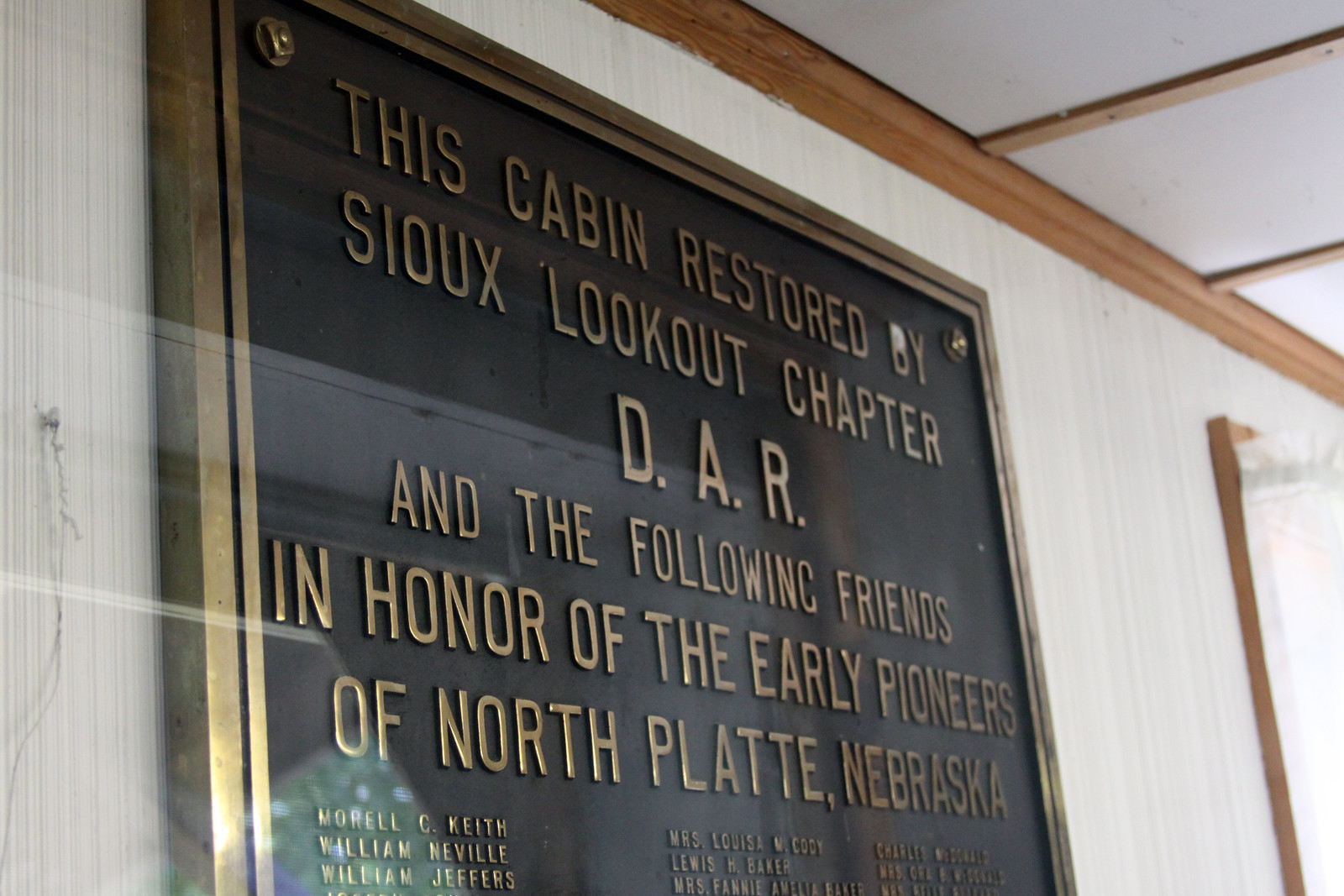This is a detailed photograph of a metal plaque mounted on a white wall, encased in a glass enclosure for protection. The plaque, which has a black background and bronzish lettering framed with bronze, commemorates the restoration of a cabin by the Sioux Lookout Chapter D.A.R. (Daughters of the American Revolution) and several friends in honor of the early pioneers of North Platte, Nebraska. The prominent text reads, "This cabin restored by Sioux Lookout Chapter D.A.R. and the following friends in honor of the early pioneers of North Platte, Nebraska." Below this dedication are names including Morell C. Keith, William Neville, William Jeffers, Miss Louisa M. Cody, Louis H. Baker, Miss Fanny Amelia Baker, and Charles McDonald, among others. The plaque is secured to the wall with bronze bolts at the top corners. The setting appears to be indoors, under a white ceiling accented with brown wooden beams.